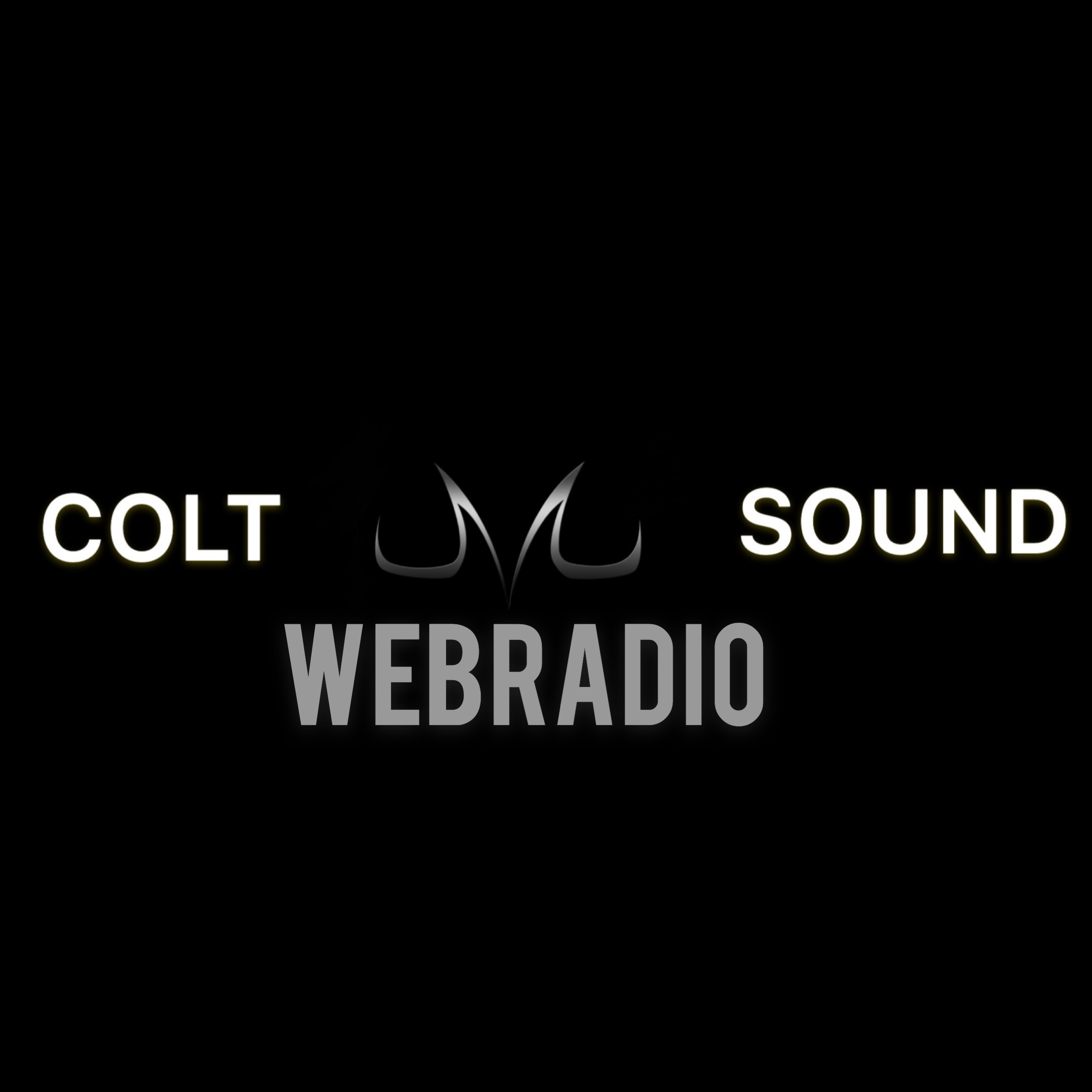The promotional media piece is a nearly square, black background featuring centrally-aligned text and a stylized logo. At the left edge of this composition is the word "COLT" in large, bold, white capital letters. Adjacent to it, in the center, is a sharp, sleek "M" rendered in a gradient gray, transitioning from bright silver to dark gray. This "M" is distinctive with its sharp, upward-curving points and a swooping base. To the right of the "M" is the word "SOUND," also in bold white capital letters, completing the top line of text. Directly beneath this top alignment, the word "WEBRADIO" is displayed in gray, uppercase letters. The entire layout is minimalistic and clean, with all elements precisely centered against the stark black background, exuding a modern and sophisticated design.